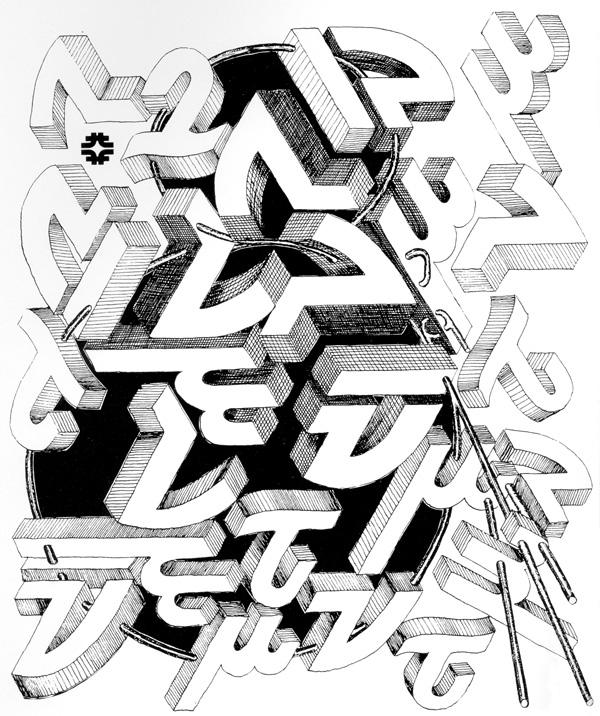The image is a detailed black and white drawing, oriented as a tall vertical rectangle slightly higher than it is wide. The drawing features an assortment of white characters that resemble abstract letters or symbols from an unrecognizable alphabet, possibly another language, jumbled together in various shapes and angles. Some of these symbols look like they could be numbers, such as the number seven, two, and possibly an upside-down two. There is also an 'N', a 'U', and an 'I', with a lowercase 'h' notable in the bottom right corner and another lowercase 'h' in the far right corner. 

These characters are scattered across a composition that includes two overlapping black circles creating a dual-circle background— a smaller circle on top and a larger one at the bottom, both intertwined with the symbols placed in front of them. On the top left corner, there's an Asian-inspired black logo and a distinct 'A' letter, depicted as a 3D shape with one leg bending towards the viewer and the other extending to the right. Additionally, this area features a curvy design made of four curves pointing towards each other with a line crossing through the sides. Elements resembling abstract poles or sticks can be seen in the corners, adding to the intricate and multifaceted design of the image.